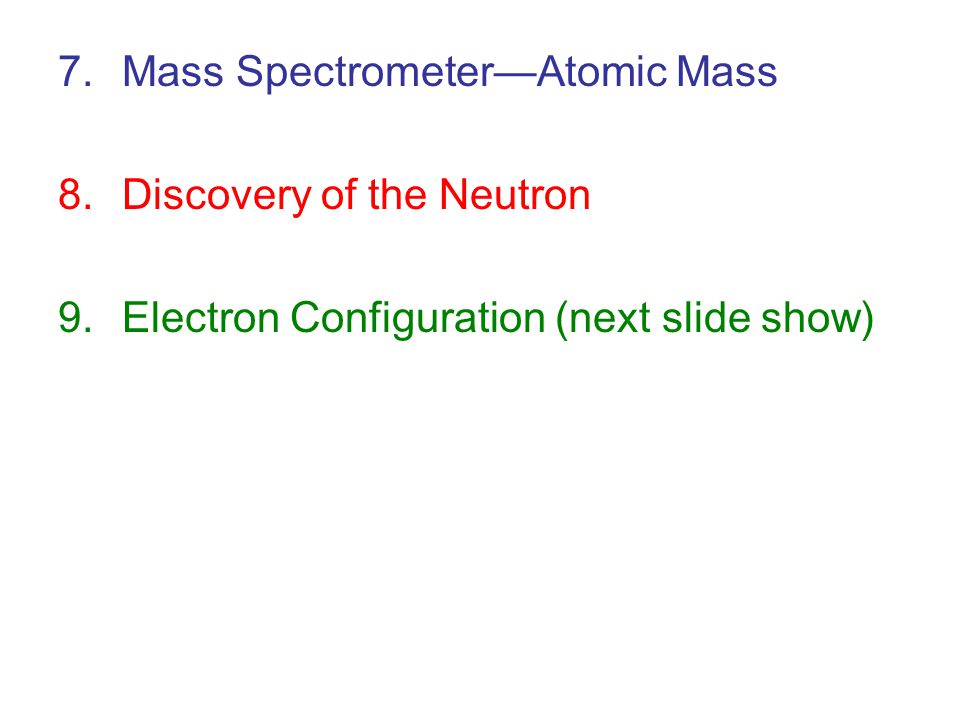The image depicts a plain white background with no borders or additional artwork, resembling a science-related lecture or presentation slide. The text is organized into three lines, each numbered and colored differently, suggesting this is an extract from a larger series of slides, likely positioned towards the middle. The first line, in blue font, reads "7. Mass Spectrometer - Atomic Mass." The second line, in red font, states "8. Discovery of the Neutron." The third line, in green font, says "9. Electron Configuration (Next Slideshow)." Each numbered item appears to correspond to key topics within a scientific lecture or slideshow presentation.